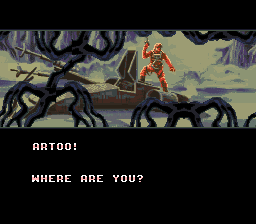This image is a screenshot from a vintage computer game, likely from the 1980s or 1990s. The screenshot itself occupies just under half of the total image area and is framed by a thick black border at the top, with a substantial, very dark black expanse beneath it. Within this black area is white text displaying, "A-R-T-O-O!" and below that, "Where are you?" 

The game image depicts Mark Hamill's character, Luke Skywalker, standing on top of his X-Wing fighter amid a dense swamp. The swamp vegetation is visible in the foreground, partially obscuring the view of the X-Wing. Additionally, the detailed swamp scenery extends into the background, enhancing the immersive setting. This classic game scene captures a nostalgic moment, indicative of early video game graphics and storytelling.